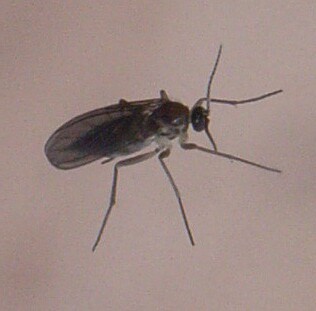This is a detailed close-up photograph of a small insect with a distinctive black body and translucent, folded wings, occupying the center of a square image. The background is a textured off-white or light brown beige color, and the image appears slightly low-resolution. The insect features a notably small, round, black head, from which extend two long, slender black antennae that curve gently outward. Its body is oval-shaped, tapering to a point at the rear but not featuring a visible stinger. The creature’s six segmented legs are also thin and black, with three visible on one side due to the insect's slight angle. The wings, though darkened slightly, remain transparent enough to reveal the body beneath them. Overall, the insect resembles a gnat or small fly but is distinct with its elongated limbs and pointed body shape.